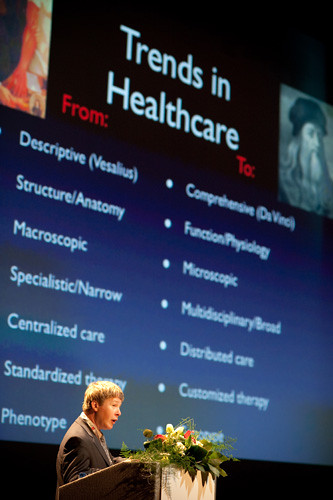The image features a man with short brown hair dressed in a dark gray business suit, standing behind a wooden podium adorned with flowers and plant leaves. Positioned centrally at the bottom of the photograph, he addresses an audience. Behind him, a large projection screen dominates the background, displaying a PowerPoint slide with the title "Trends in Health Care" at the top. The slide is organized into two columns. The left column, labeled "from," lists terms such as "descriptive structure/anatomy," "macroscopic," "specialistic/narrow," "centralized care," "standardized therapy," and "phenotype." The right column, labeled "to," transitions these terms to "comprehensive (da Vinci)," "function/physiology," "microscopic," "multidisciplinary/broad," "distributed care," and "customized therapy." The setting is brightly lit, enhancing the clarity of the image.